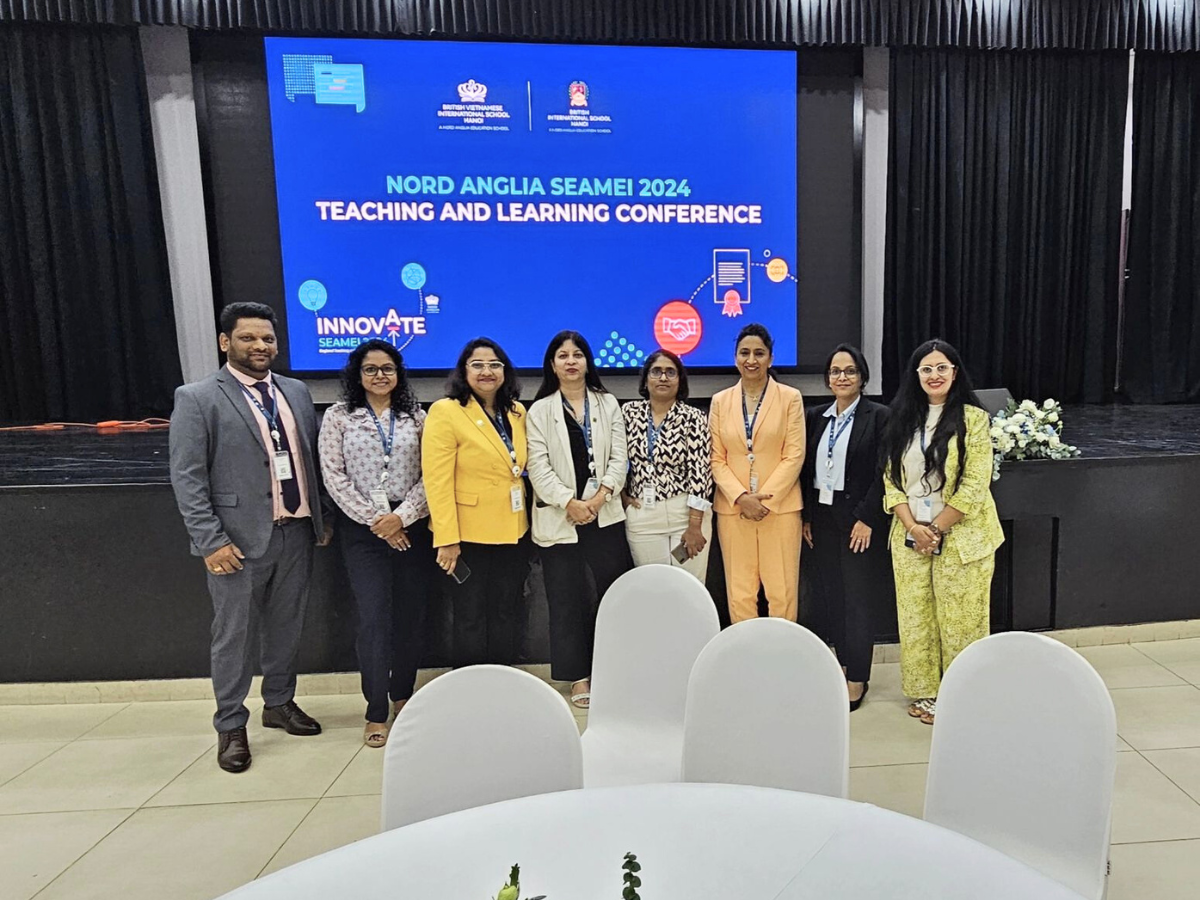The photograph, captured indoors, is a rectangular 6-inch wide by 4-inch high image featuring a group of predominantly middle-aged people of Middle Eastern or Indian descent. Positioned centrally in the room, they stand in front of a raised black stage adorned with matching curtains. A blue presentation screen at the center of the stage displays the text "Nord Anglia SEAMEI 2024 Teaching and Learning Conference" in white, with additional design elements and arrows possibly pointing to the word "Innovate."

At the bottom of the image, large cream-colored square tiles cover the floor. In the foreground, a round table with a white tablecloth and matching white chairs is partially visible. The group consists of one man, located on the far left, wearing a gray suit, dress shirt, tie, and lanyard, with dark black hair and a finely trimmed beard and mustache. The remaining seven individuals are women dressed in various forms of office attire, each also wearing lanyards. They all have light brown skin and dark black hair, which varies from straight to slightly curly.